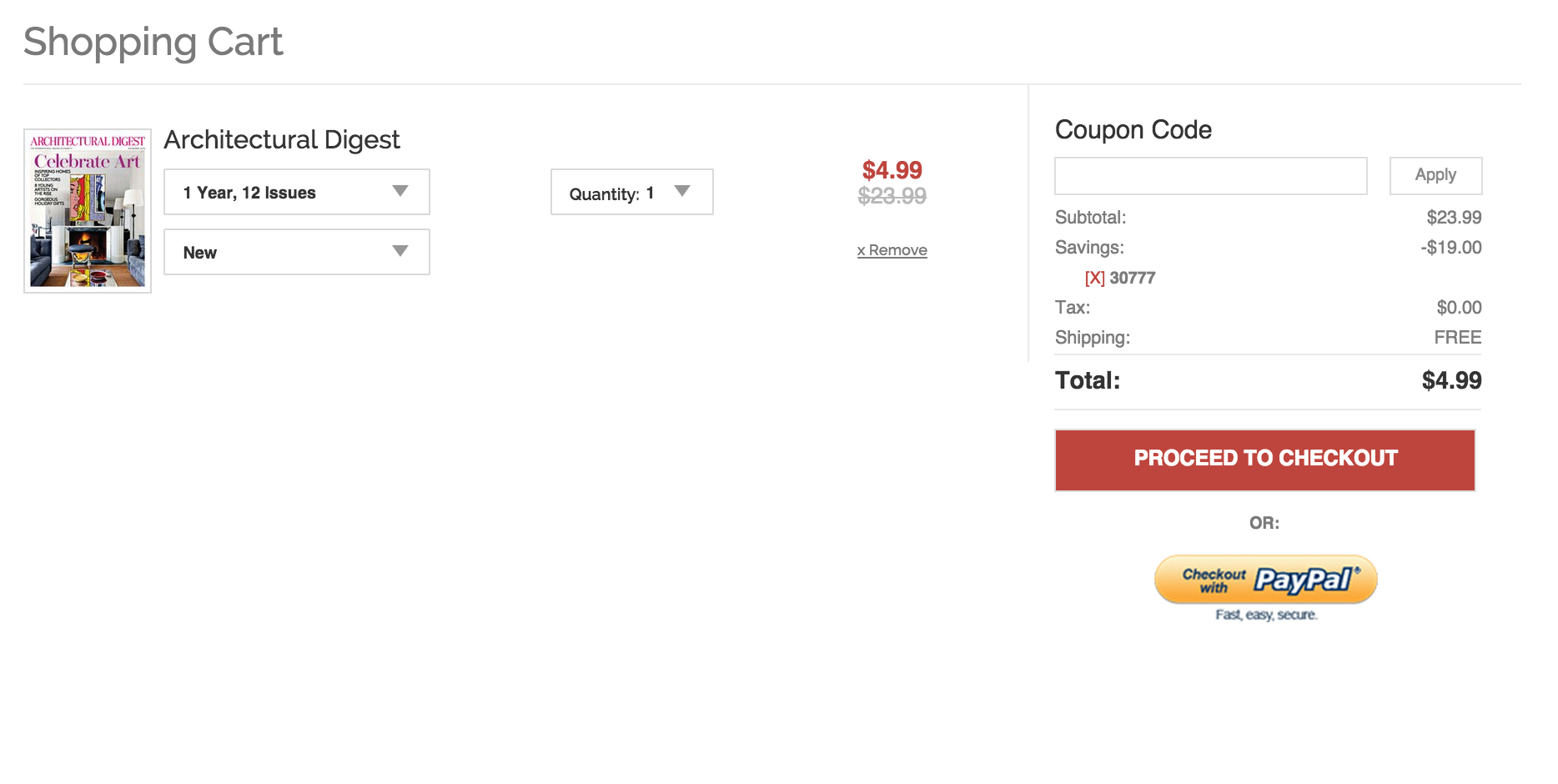The screenshot captures the top left portion of a web page displaying an online shopping cart for an art publication. The header includes a gray icon labeled "shopping cart," followed by the phrase "Celebrate Art" next to a white desk. Displayed are various art pieces in red, yellow, blue, and white. Bold black text reads "Architectural Digest," accompanied by two dropdown menus. 

The first dropdown, "One year, 12 issues," features a gray dropdown triangle. The second dropdown labeled "New" also has a gray dropdown triangle. In the center, the item quantity is set to one in bold black text with another gray dropdown arrow. To the right, red text displays the discounted price of $4.99, with the original price of $23.99 crossed out in gray beneath it. Below, a black-lined option reads "X Remove."

On the right-hand side, a small rectangle divided by a line features a bold black "Coupon Code" label. There is a blank rectangle meant for entering a coupon code alongside a black "Apply" button. Below, black text displays the subtotal as $23.99 with savings of $19. A red "X" shows a code "30777," and further details indicate zero tax and free shipping, leading to a total of $4.99.

At the bottom, there is a red button with bold white text stating "Proceed to Checkout," followed by the word "or." A gold circular button offers the option to "Check out with PayPal" in white text within a blue border. The footer text reads "Fast, easy, secure" in black.

This image provides a detailed view of an online subscription purchase interface for "Architectural Digest," emphasizing discounts, coupon code entry, and multiple checkout options.